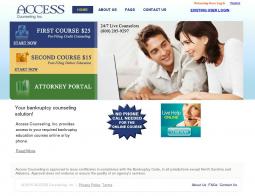A low-resolution screenshot from the Access website, which appears to be a consulting firm, shows a man in a white button-down shirt and a woman in a white t-shirt looking at a laptop. Beside them is a text phrase promoting "24-7 live conversation" followed by an illegible phone number due to the small text size. The top navigation bar features several tabs, including "About Us," "Press," and "Contact Us." Opposite the individuals, there are various buttons stating "First course $25," "Second course $15," and "Attorney Portal." Additional readable text on the page includes "Your bankruptcy counseling solution," as well as a partial statement, "No phone call needed for ..." The overall image quality is poor, making finer details difficult to discern.